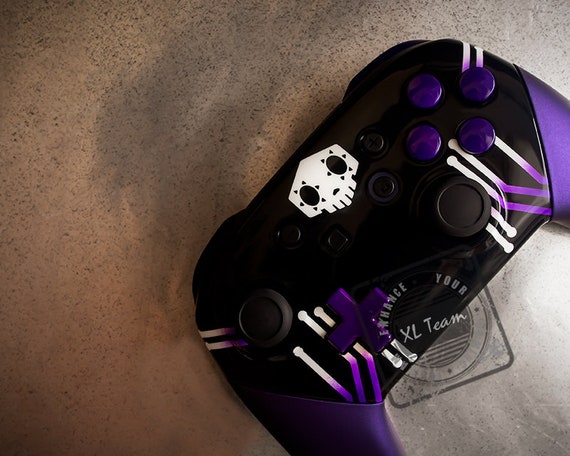This photograph showcases a custom Nintendo Switch pro controller with a distinctive Overwatch Sombra theme. The controller is predominantly purple with black accents and features a prominent white half-skull design at the top center. Positioned vertically, the controller’s two purple handles extend diagonally across the image, with one pointing towards the lower left and the other towards the upper right. The left side of the controller hosts a black joystick above a purple D-pad, both marked with white and purple stripes. On the right side, there is another black joystick located just below a cluster of four purple buttons. Additional details include subtle white lines that blend into purple on the handles. The background appears to be a speckled concrete surface, and a watermark reading "Enhance Your Gaming XL Team" is present.